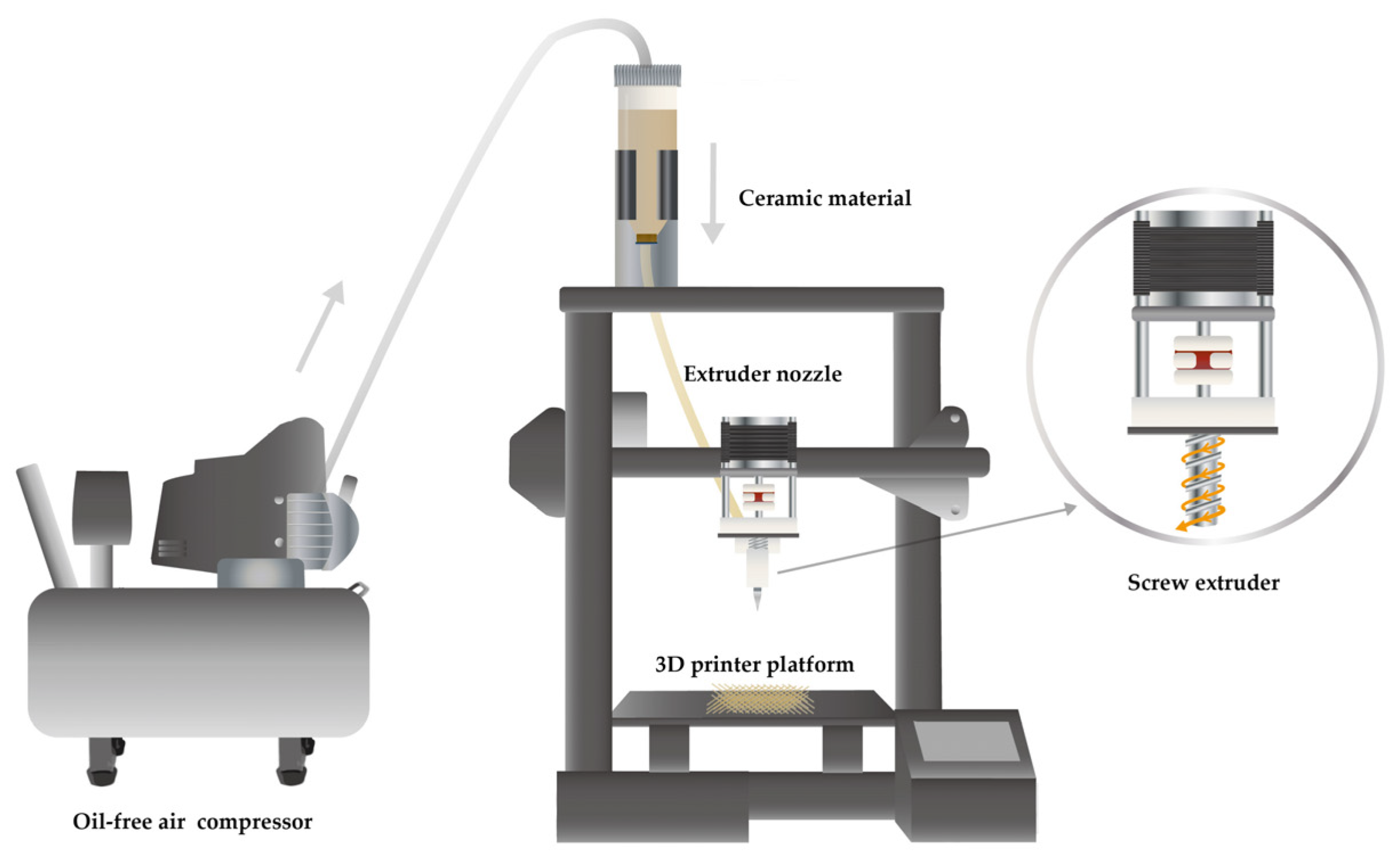The image is a detailed diagram illustrating the various parts of a 3D printer on a white background, presented in a side view arrangement. At the center is a square box labeled "3D Printer Platform" in black text. Positioned above the platform is a small square box containing a red element, which is identified as the extruder nozzle. A close-up inset highlights the screw extruder situated beneath the red screw-like component. Additionally, above the extruder nozzle, there is a cone-shaped object labeled "Ceramic Material." To the left side of the diagram, there's an oil-free air compressor depicted as a gray rectangle with short legs. This compressor is connected by a hose that runs up to the ceramic material, with an indication of how the compressed air facilitates the movement of the ceramic material through the extruder nozzle to produce prints on the 3D printer platform. The diagram also features textual annotations and directional arrows that enhance the understanding of the printer’s operation, with the overall illustration style reminiscent of Adobe Illustrator, employing simple shapes with subtle gradients.